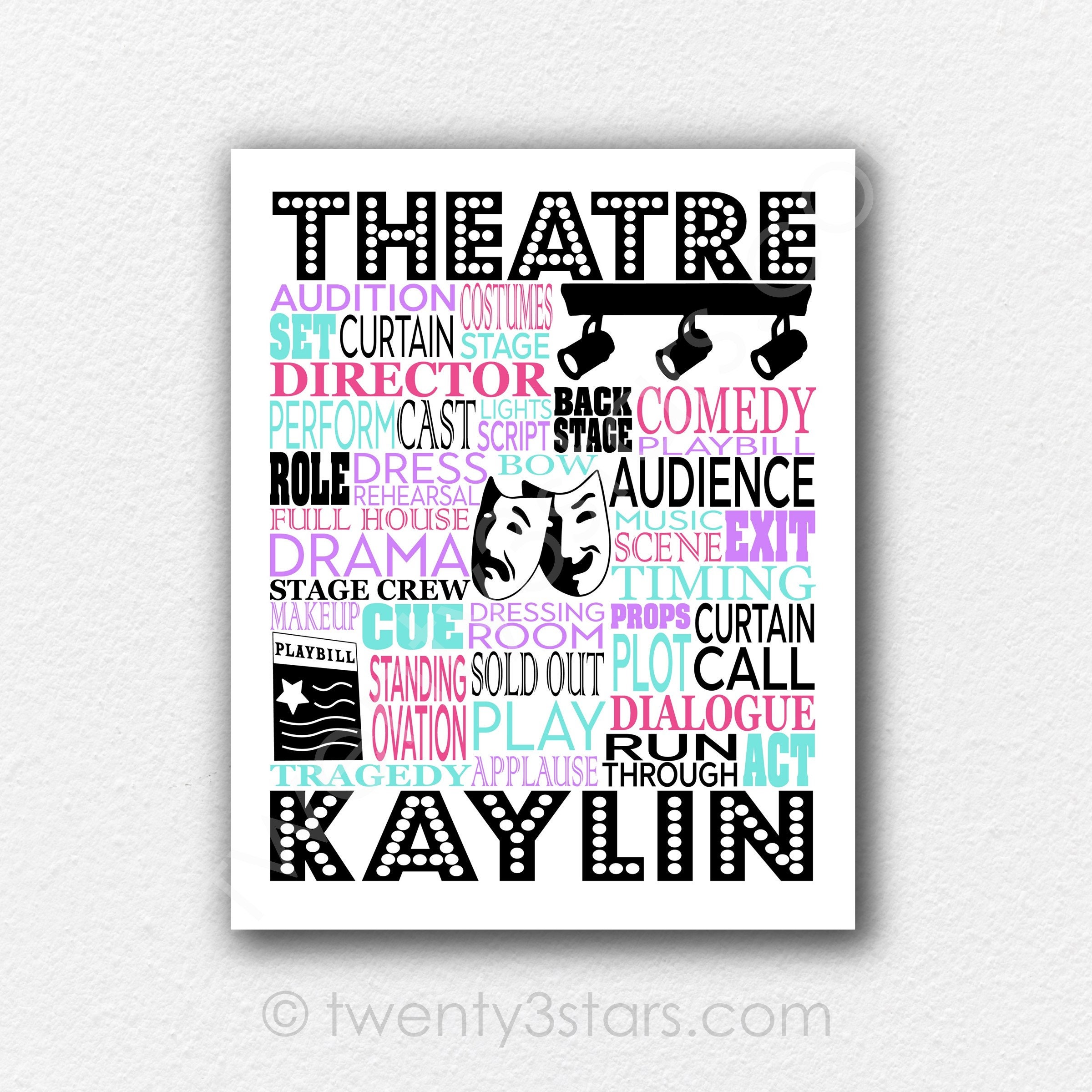This image depicts a vibrant theater-themed poster prominently featuring the text "Theater KAYLIN" at the top and bottom. The centerpiece of the design is a classic pair of comedy and drama masks, symbolizing theatrical art. Surrounding them is a colorful word cloud composed of terms related to theater, including "audition," "costumes," "script," "curtain," "stage," "director," "comedy," "drama," "audience," "backstage," "playbill," "stage crew," "standing ovation," "sold out," "run through," "dialogue," "act," "applause," "tragedy," "bow," "lights," "set," "perform," "rehearsal," and "schoolhouse." These words are displayed in a variety of colors such as red, green, purple, black, pink, and baby blue against a white background. The image, which has the appearance of a real photograph, is set against a textured white wall and includes a watermark that reads "copyright 23stars.com" at the bottom.